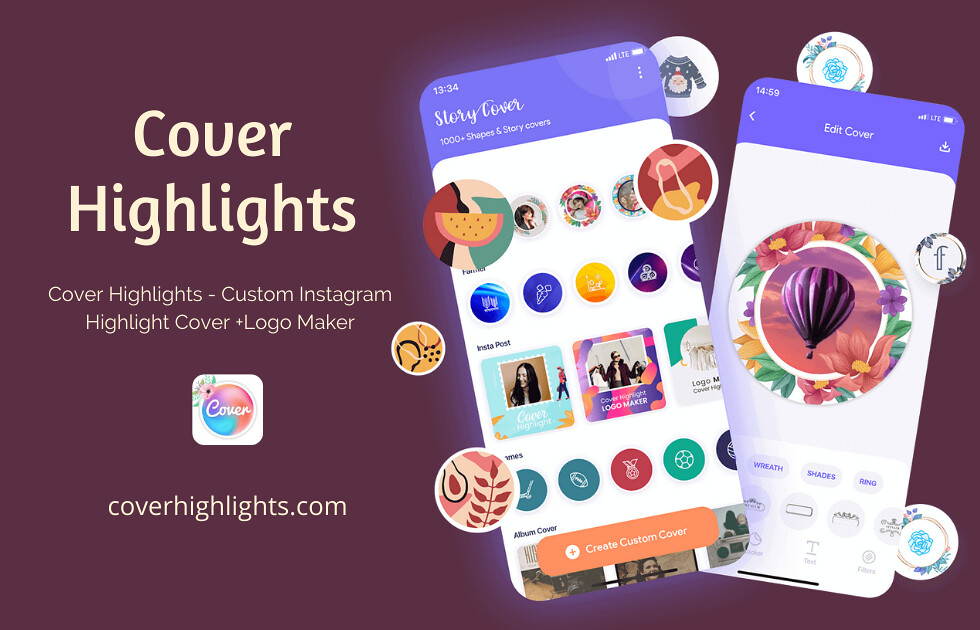The image is an advertisement for an app designed to create custom Instagram highlight covers and logos. The background is a rich burgundy color. On the left-hand side, it prominently displays the text "Cover Highlights" in a light, off-white yellow color, followed by "Custom Instagram Highlight Cover Plus Logo Maker." Beneath this text is a square icon with a circle in the middle that features a gradient blend of blue, purple, pink, and orange, with the word "cover" inscribed. Below the icon, the website "coverhighlights.com" is listed. On the right-hand side, there are two overlapping screenshots showcasing the app's interface. One of them highlights a circle with a hot air balloon surrounded by buttons for editing, while the other displays a range of different graphics available for use. The screenshots are colorful, featuring various shapes, story covers, and icons, such as a hot air balloon with flowers and a fruit resembling a watermelon, emphasizing the app's versatility in designing covers.